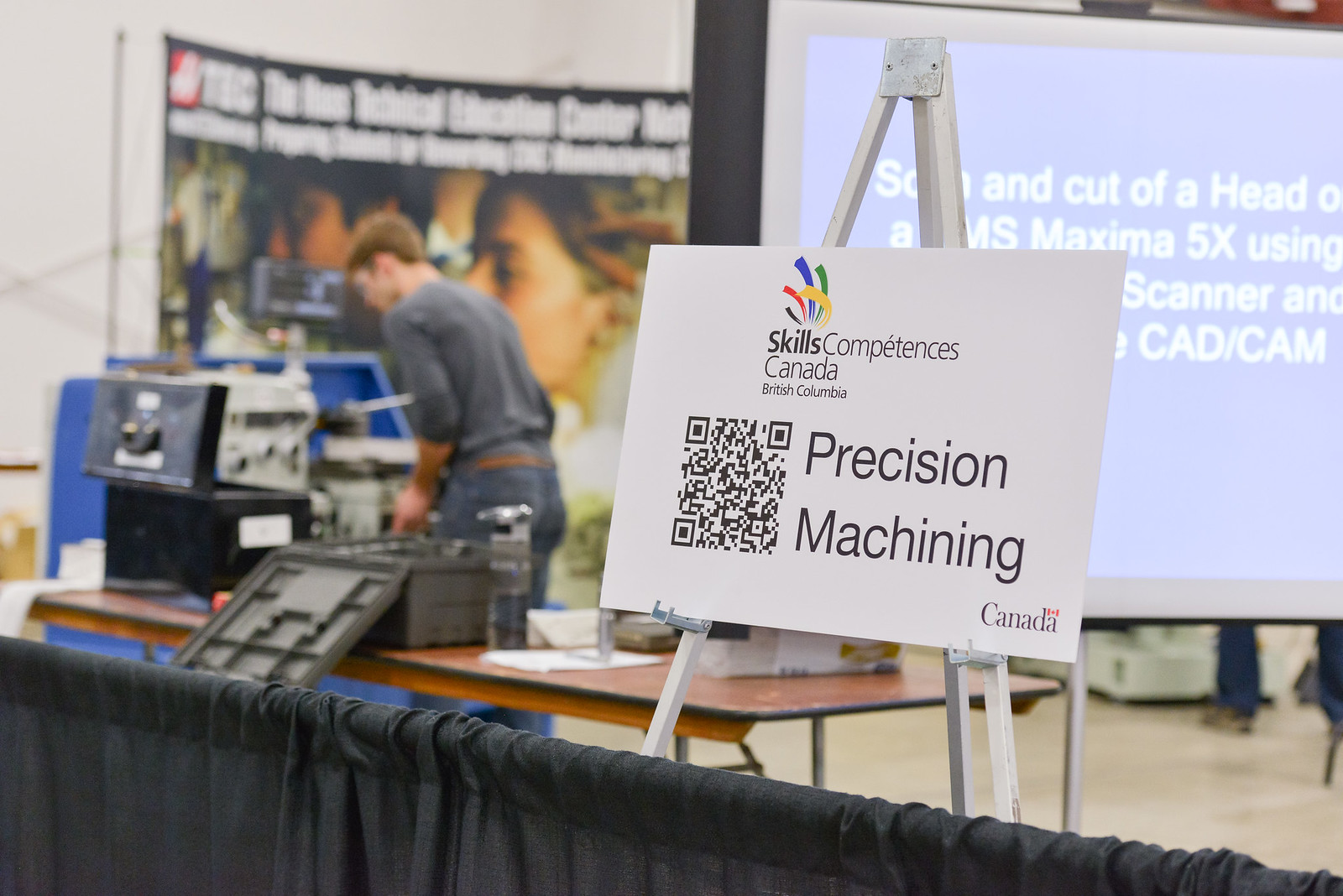The photograph captures a busy scene, likely at a science or job fair convention. Dominating the foreground is a white sign on a steel tripod stand, displaying a colorful logo with red, blue, green, and yellow lines reminiscent of fireworks. The text on the sign reads "Skills Competences Canada, British Columbia" and "Precision Machining Canada," accompanied by a QR code and the Government of Canada logo in the bottom right corner. In the background, set against a black curtain barrier, a man with dirty blonde hair, wearing a grey long-sleeved shirt with rolled-up sleeves, denim jeans, and a brown belt, is engrossed in operating machinery displayed on wooden tables. Additional equipment and a water bottle are scattered on the tables, suggesting preparations for a presentation. Large projector screens behind him partially display the text "Cut Off Ahead, Maxima 5X Scanner," hinting at a technical demonstration in progress or forthcoming.